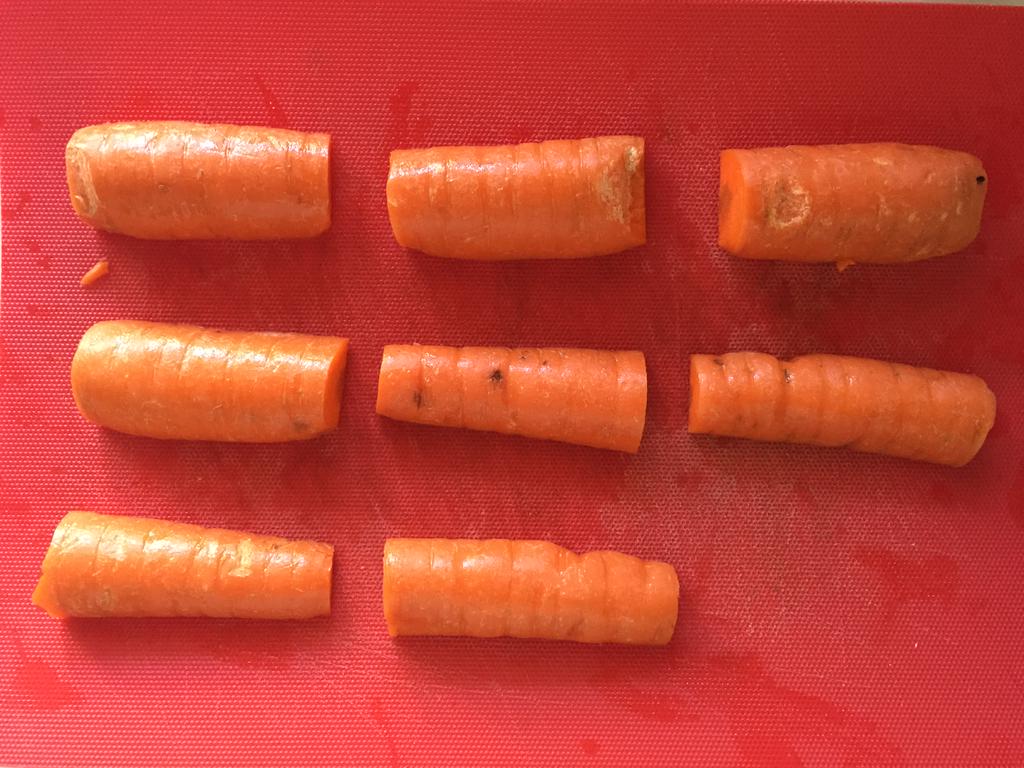This color photograph showcases eight carrot slices arranged on a textured, reddish-orange surface, likely a red silpat mat or cutting board. The carrots have been halved lengthwise and then sliced into segments, resulting in eight pieces arranged in three rows: three slices in the top row, three in the middle, and two in the bottom row on the left side. The carrots are a dark orange hue with distinctive markings and blemishes, indicating they haven’t been peeled. Each slice reveals a slight highlight moving from left to right across their flat surfaces. The textured background shows faint lines, possibly knife markings, adding to the functional and slightly worn appearance of the mat.